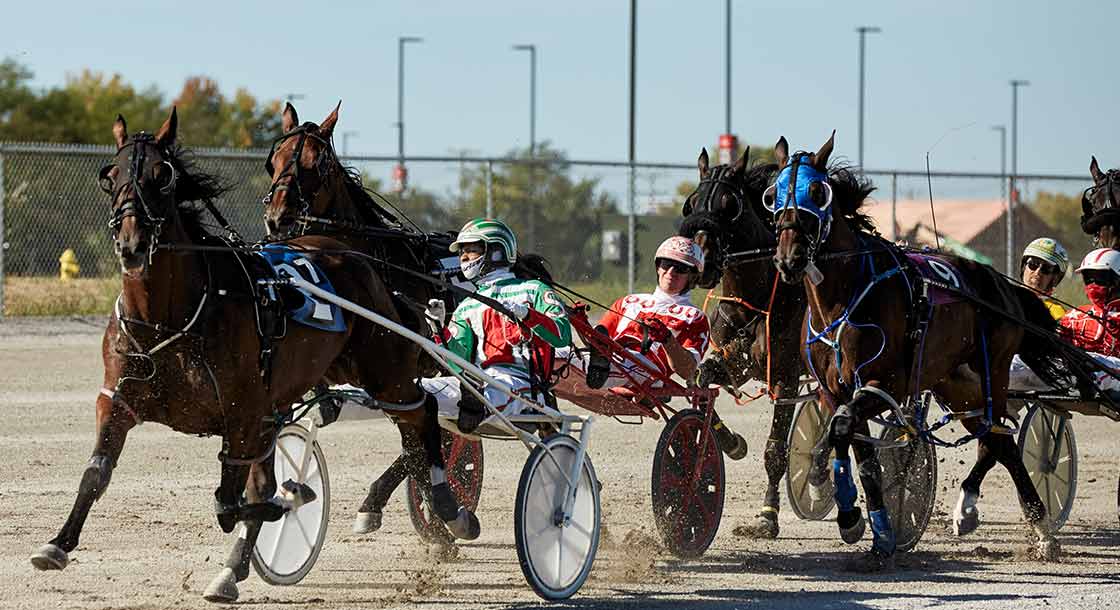In this image, a clear blue sky forms the backdrop for a vibrant scene at a modern-day horse race, reminiscent of a chariot race. Foregrounded are four horses, mostly brown with variations of black and brown markings, each adorned with colorful saddles and masks. The front horse, distinguished by its black mask and blue saddle marked with a white '07,' pulls a white carriage with matching wheels. Its jockey wears a striking outfit of white pants, a multicolored white, green, and red shirt, and a matching helmet. To the left, another horse, also in a black mask, pulls a red carriage with black-tired wheels, steered by a jockey dressed in a coordinated red and white ensemble. Two more horses, one in a black mask and the other in blue, pull their respective carriages; the latter features a purple saddle marked with '09.' Their jockeys sport yellow and white, and red and white attire, respectively. The ground at the front of the image appears muddy with tan and brown hues, while the background showcases a silver chain-link fence, tall streetlights, and lush trees. A yellow fire hydrant stands to the left amid the green-yellow grass, completing the picturesque portrayal of this exhilarating race.